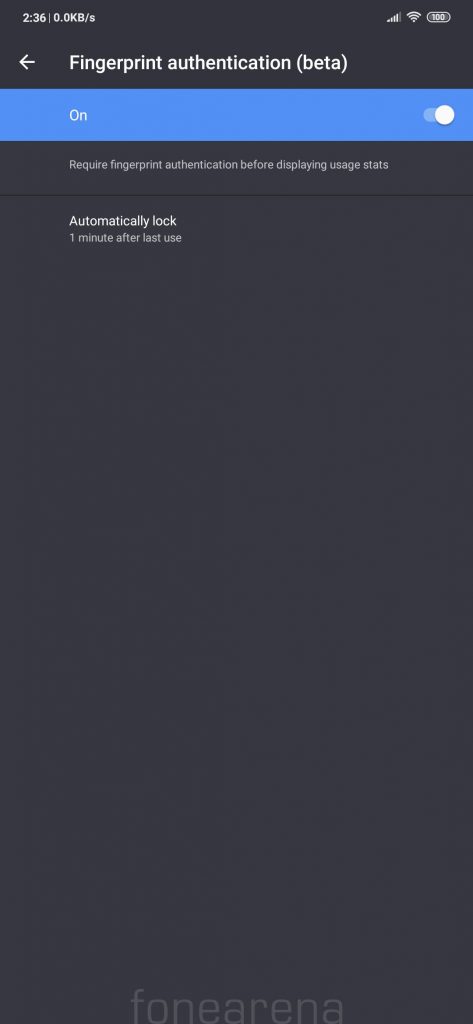Screenshot of a Phone Displaying Fingerprint Authentication Settings:

At the very top of the screenshot, there's a black bar displaying device status information in white text. On the right side, the time is shown as 2:36, followed by a data usage indicator showing 0.0 KB/s. Further to the right, a series of icons depict four cellular signal bars, a Wi-Fi symbol, and a 100% battery indicator.

Below the status bar, a large white text header reads "Fingerprint Authentication (Beta)," with a right-facing arrow icon next to it. Just beneath this, a toggle switch feature is displayed. The left side of the toggle features the word "On" in white text against a small blue bar, indicating that the fingerprint authentication is currently enabled.

Following the toggle switch, a descriptive configuration reads: "Require fingerprint authentication before display and usage stats." This text is in standard white font and is followed, after a small space, by another configuration option: "Automatically lock one minute after use," which is presented in a slightly larger font.

At the very bottom of the screenshot, a label in grayscale reads "Phone Arena," likely indicating the name or brand associated with the application or settings interface.

The overall color scheme is predominantly black and white, with occasional blue accents for the toggle switch, creating a minimalistic and functional design for the fingerprint authentication settings screen.